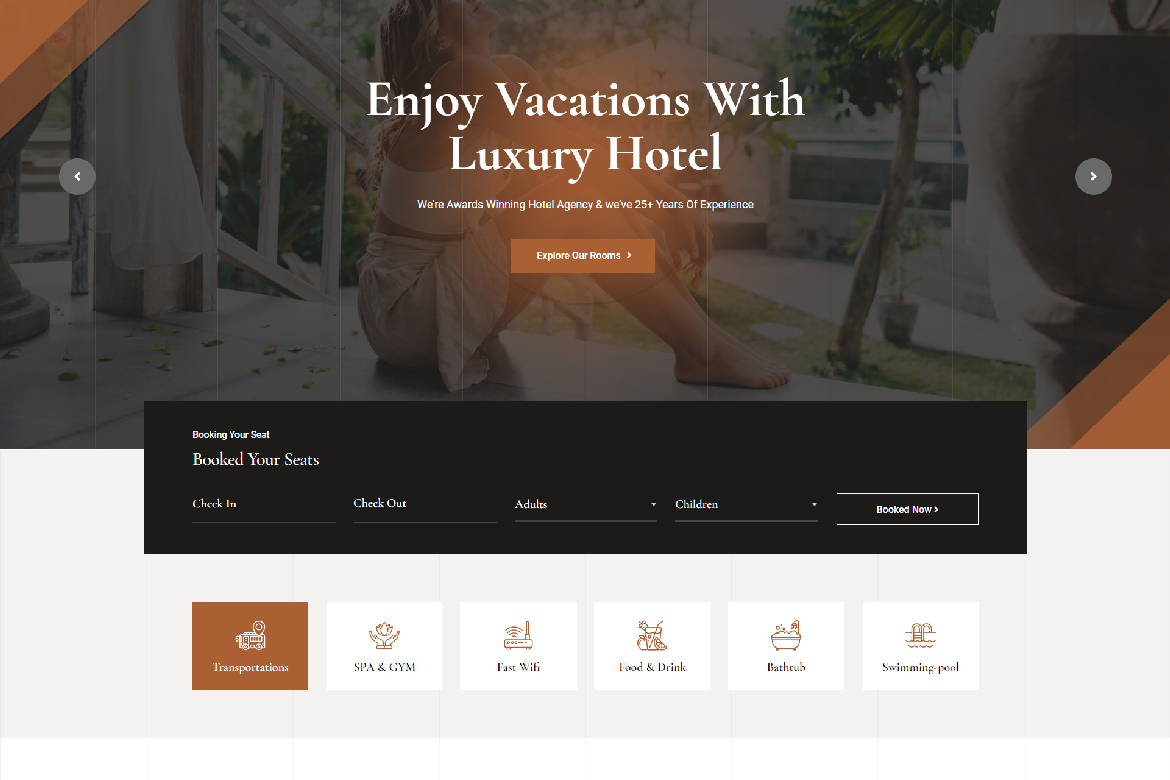The image features an advertisement banner at the top that reads, "Enjoy Vacation with Luxury Hotel" in white text. The photograph beneath has a dark gray tint, making fine details indistinguishable. It depicts a woman sitting on a porch. She is barefoot and wears a shoulderless dress. Her knees are drawn up to her chest. Surrounding her in the background are trees, a concrete walkway, and some potted plants. 

Below the image, there is a small black box that is difficult to read due to its size. However, it does contain fields labeled "Check-In" and "Check-Out," with a button visible for submission of that information. Underneath this black box, there are six smaller boxes set against a gray background, each highlighting different amenities: Bar and Gym, Free Wi-Fi, Food and Drink, Breakfast, and Swimming Pool.